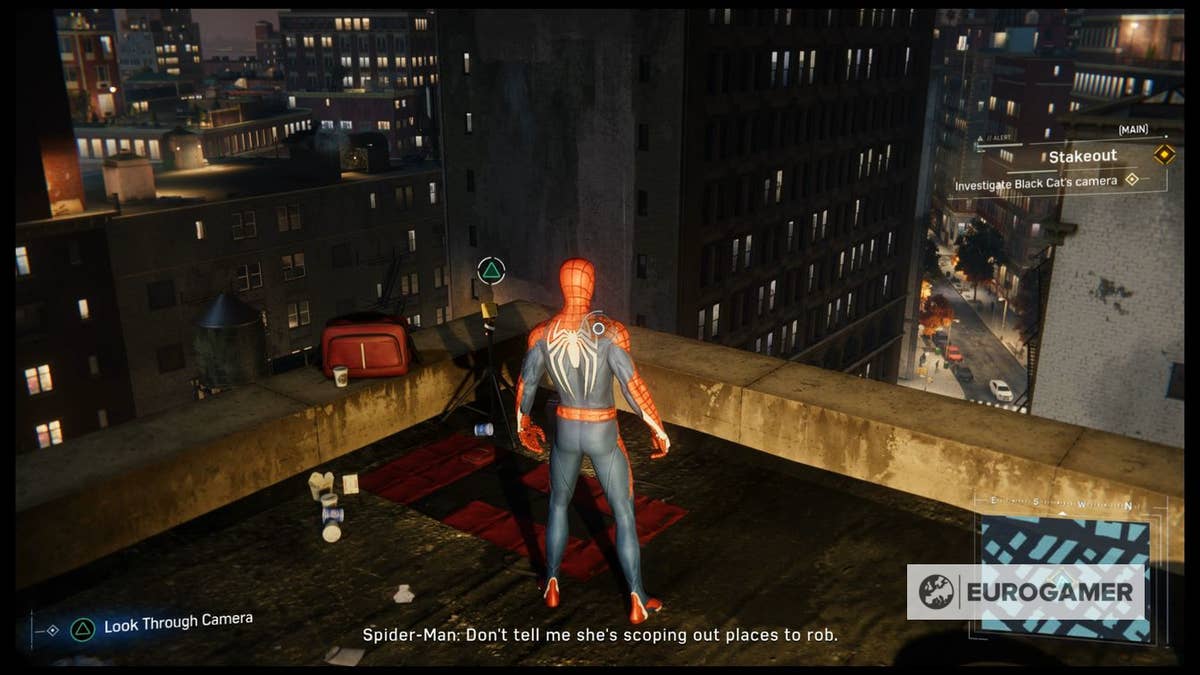The screenshot from the Spider-Man video game captures a vivid scene where Spider-Man, in his iconic red and blue suit emblazoned with a white spider on the back, stands on the rooftop of a tall building. He looks down upon a sprawling, brightly lit cityscape that closely resembles New York. Apartment buildings abound with glowing windows and cars move along the streets far below. In front of Spider-Man is an interactive telescope highlighted by an icon with a triangle button prompt, encouraging the player to use it. The game's interface overlays the image, with text at the bottom center reading, "Spider-Man: Don't tell me she's scoping out places to rob" and in the top right corner featuring a mission detail: "Main Stakeout - Investigate Black Cat's camera." The game’s publisher, Eurogamer, has its logo displayed prominently in the bottom right corner. The overall clarity of the image is sharp, capturing a bright and detailed urban environment.